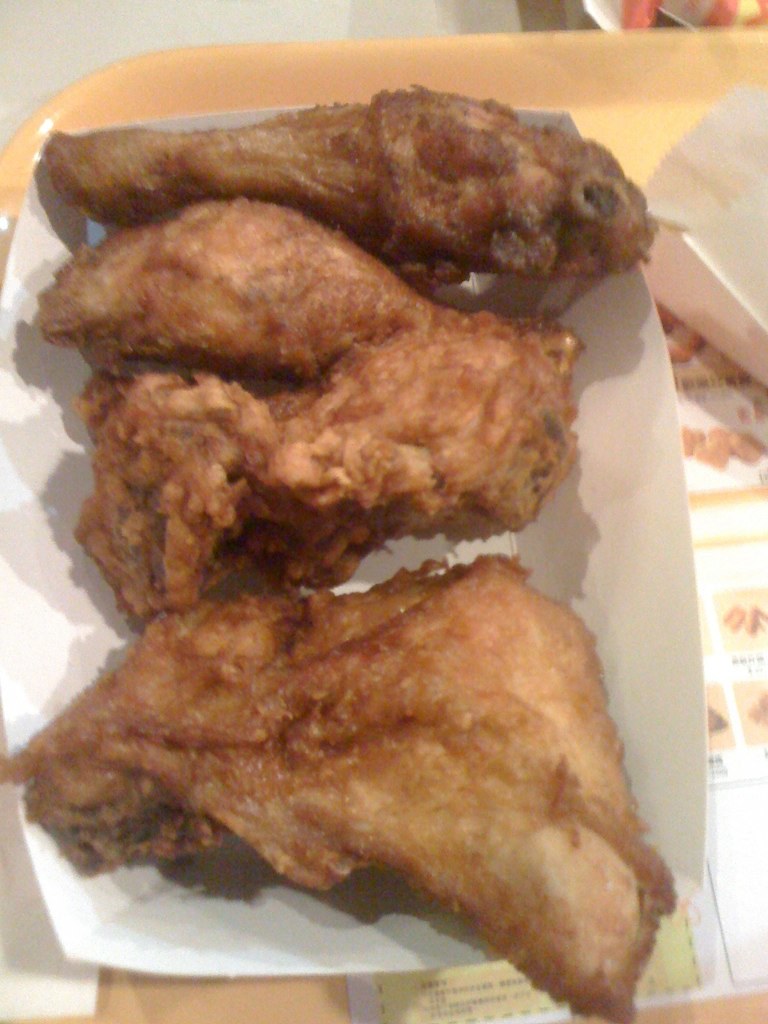This photo depicts a plastic takeout tray featuring an open white paper carton filled with four pieces of golden-brown fried chicken, each piece distinctly on the bone. The chicken pieces include two drumsticks at the top, which are notably skinny, and two larger pieces that resemble wings. The carton thoroughly contains the chicken, emphasizing its substantial quantity. Underneath the carton, a cream-colored paper advertisement or menu is partially visible, adorned with indistinct pictures of food. A small white takeout bag, possibly intended for fries, is placed to the top right of the carton, all arranged neatly on the plastic tray.